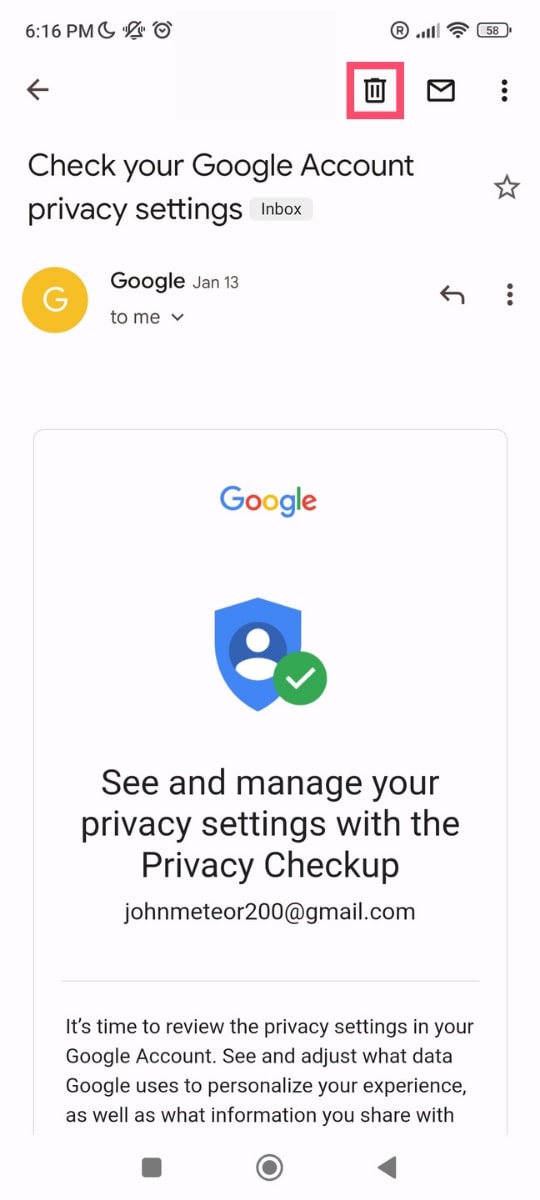A screenshot of an email sent by Google on January 13th invites the recipient, identified as JohnMeteor200@gmail.com, to review their Google account privacy settings. The email, titled "Check your Google account privacy settings," features a shield icon for security and prompts the recipient to "See and manage your privacy settings with the Privacy Checkup." It emphasizes the importance of adjusting and personalizing privacy settings to enhance their Google experience.